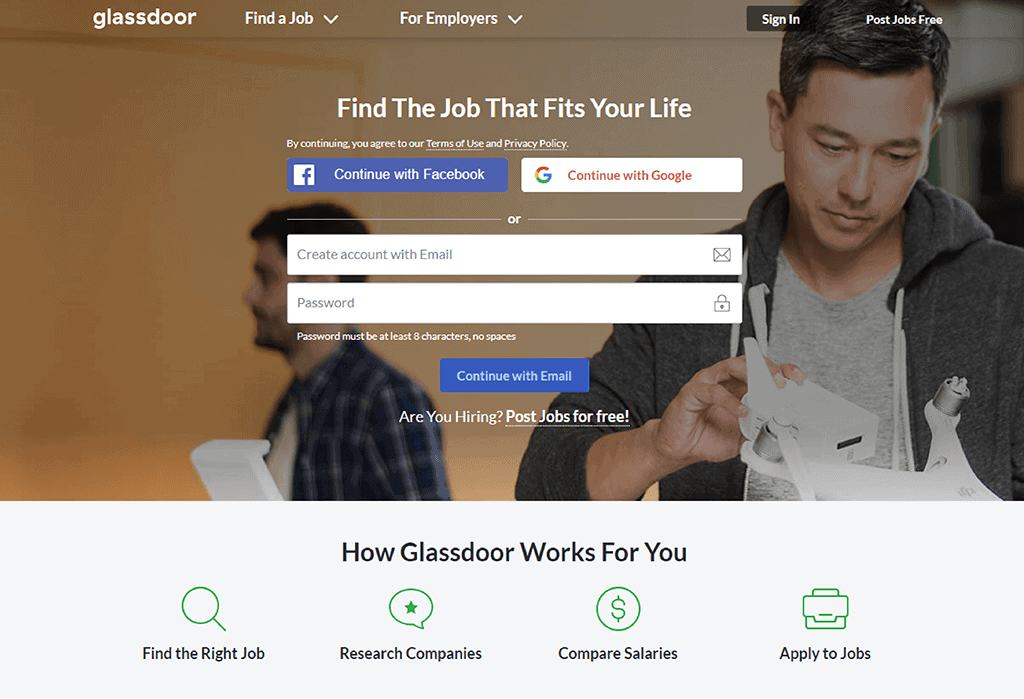A screen capture from the Glassdoor website illustrates its login page. At the top of the page, a white header features the Glassdoor logo on the left, followed by navigation options: "Find a Job," "For Employers," "Sign In," and "Post Jobs Free."

The central area of the page showcases a background image of two individuals. On the right, a young man, approximately 25 to 30 years old, is focused on a small toy drone. He appears to be adjusting something on the drone, with a tool or remote in his right hand.

Overlaying the image is a prominent white text that reads, "Find the job that fits your life." Directly below, the login options are displayed with logos for Facebook and Google indicating "Continue with Facebook" and "Continue with Google" respectively. An alternative login method allows users to "Create Account with Email," accompanied by a field for password entry. 

At the bottom of the page, a prompt states "Continue with Email" alongside an invitation for employers: "Are you hiring? Post Jobs for Free."

Further, a gray ribbon at the bottom outlines additional resources. From left to right, headings read "Find the Right Job," "Research Companies," "Compare Salaries," and "Apply to Jobs," each paired with a green icon. Above these headings, the text "How Glassdoor Works for You" summarizes the section's purpose.